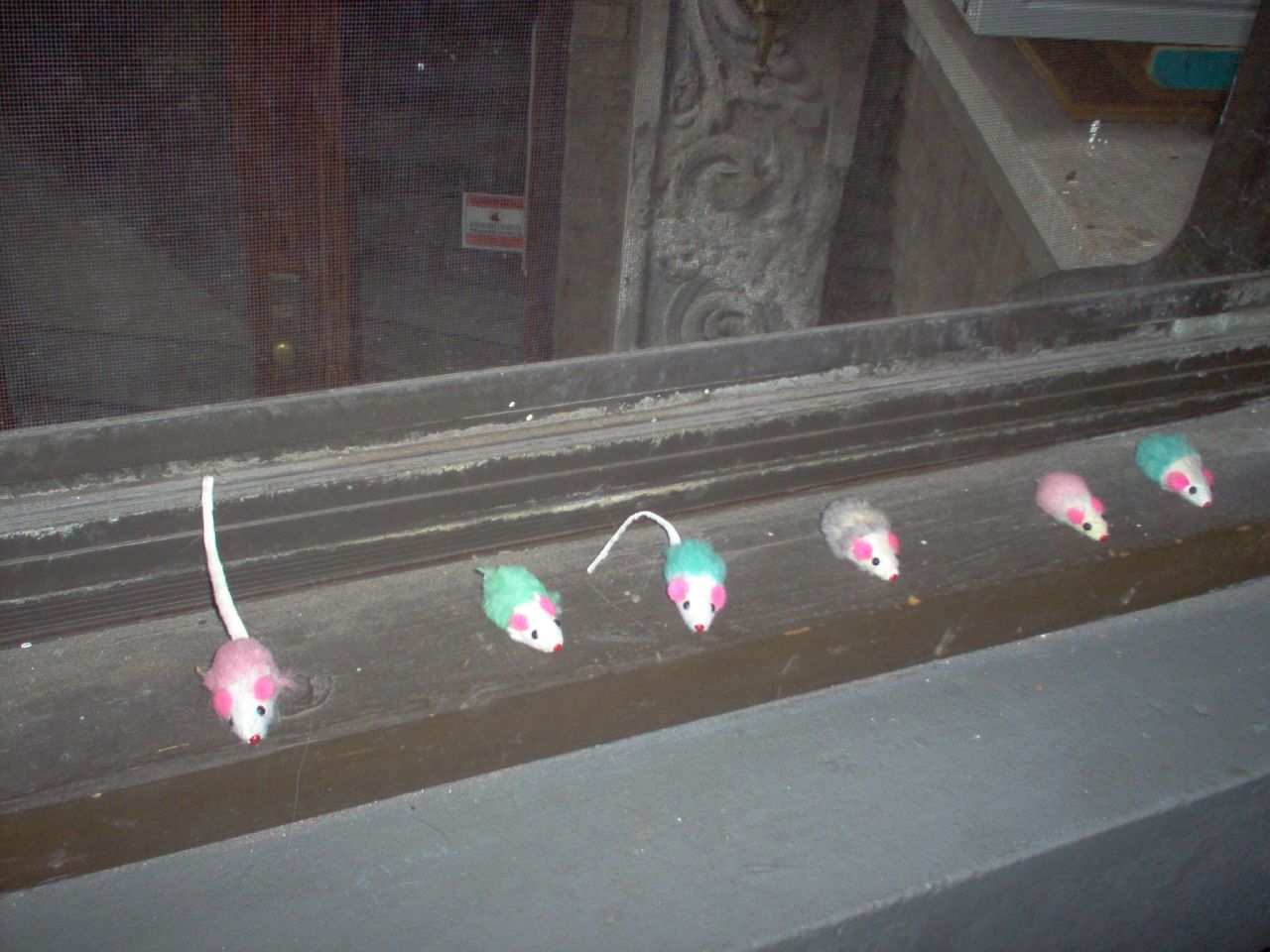The photograph captures a dusty, dark brown wooden windowsill lined with six small, stuffed catnip mice arranged in a row. The windowsill, which looks aged and grimy, sits in front of a window track covered in dust. Each of the toy mice features pink ears and a white face, but their bodies vary in color and orientation: the first is pink and facing the camera, the second is green and white facing slightly right, the third is green and white facing directly forward, while the fourth, fifth, and sixth are gray, pink, and dark green, respectively, all facing slightly right. Visible through the window is a glass door, adorned with a brass handle and a possible neighborhood watch warning sign, set within a relief-carved frame, resembling either stone or wood. The indoor scene includes a short, dingy white wall beneath the windowsill, with some parts capped in marble. The area gives off a sense of being part of an old building, possibly an apartment unit.